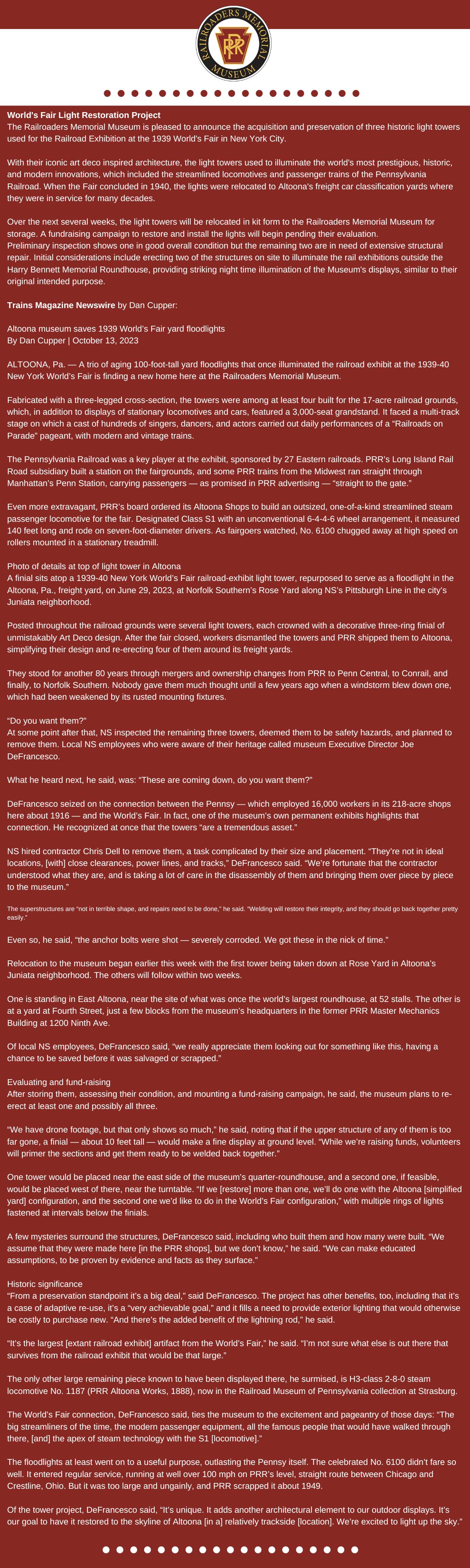The image shows a large, red rectangular document that is covered in small, illegible white text. At the top of the document, there is a white area featuring a medallion in the center. The medallion contains a portion of the red background with three yellow letters, "HFR," which are the only legible part of the document. This medallion is encased in a black circle that also has illegible lettering around its perimeter. The document appears to be very lengthy, potentially an infographic or informational text, and concludes with several white circles lining the bottom, implying the possibility of navigation dots for additional content. The overall design suggests the document could be related to a college, featuring a seal with a prominent keystone element. The intricate layout and illegibility indicate it might be a high-detail image where vital information, facts, or rules are presented in very small text.